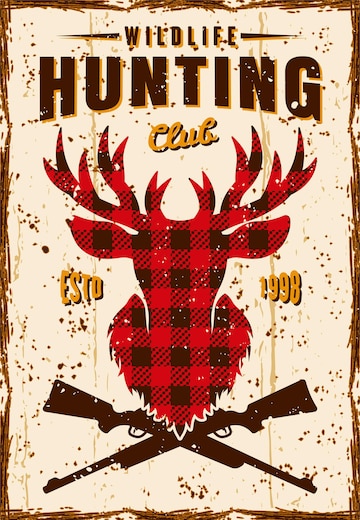The poster for the Wildlife Hunting Club, established in 1998, prominently features the club's name at the top. "Wildlife" and "Hunting" are written in dark brown letters with an orangish shading around them, while "Club" is in an orange cursive font. Centrally, a flannel-patterned deer head with antlers, rendered in a red and black plaid design, draws immediate attention. Below the deer head, two brown rifles are crossed in an X pattern, evoking a skull and crossbones motif. The words "ESTD" and "1998" flank the deer head, written in orange. The poster itself has a lighter brown or cream background with darker brown speckles and is bordered by a darker brown edge, adding a rustic touch to the overall design.